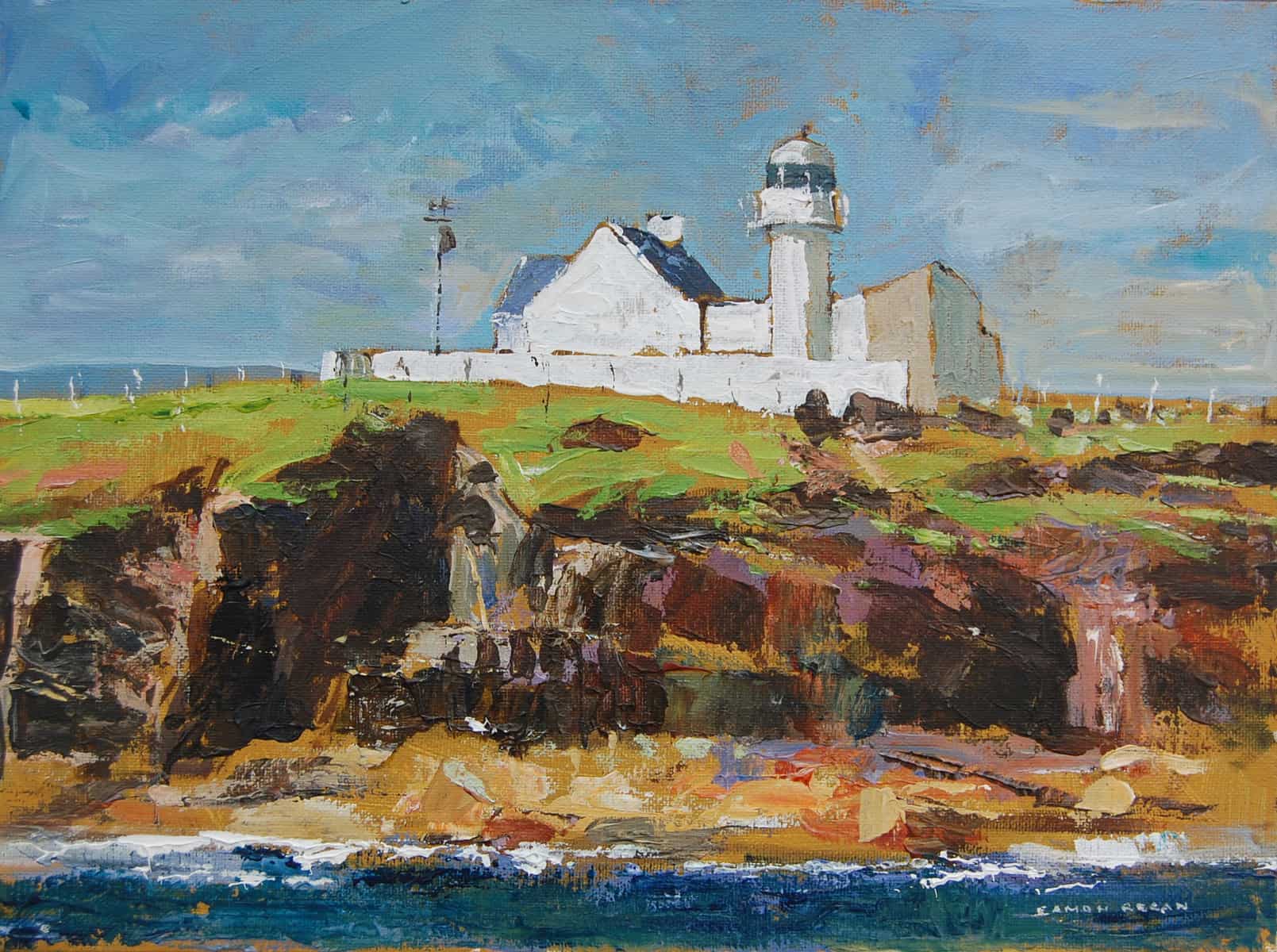This painting portrays an impressionist-style watercolor scene of a coastal lighthouse complex situated on an island. The artwork is characterized by sharp, chisel-like brushstrokes that create a striking texture typically unusual for watercolors. The overall composition is in a wide vertical rectangular format, set during daytime, with a radiant blue sky painted with soft clouds at the top and blue ocean waves cresting against a sandy beach with jagged, earthy brown rock formations in the foreground.

In the mid-ground, patches of green and brown grasses emerge, blending seamlessly into the rocky shoreline. Perched on the high grounds of this rocky tundra is a white stucco building with a distinctive blue triangular roof, consistent across the various descriptions. The building is complemented by a tall, white cylindrical lighthouse with blue windows encircling its top, and a blue stripe around its summit. 

Adjacent to the lighthouse on the grounds stands a windmill or weather vane, depicted as a steel pole with a horizontal element at its peak. A white fence encircles the house and lighthouse, adding to the quaint, structured appearance of this coastal sanctuary. The scene is beautifully balanced between the contrasting colors of the rocky earth, the lush grasses, and the serene blues of the sky and sea.